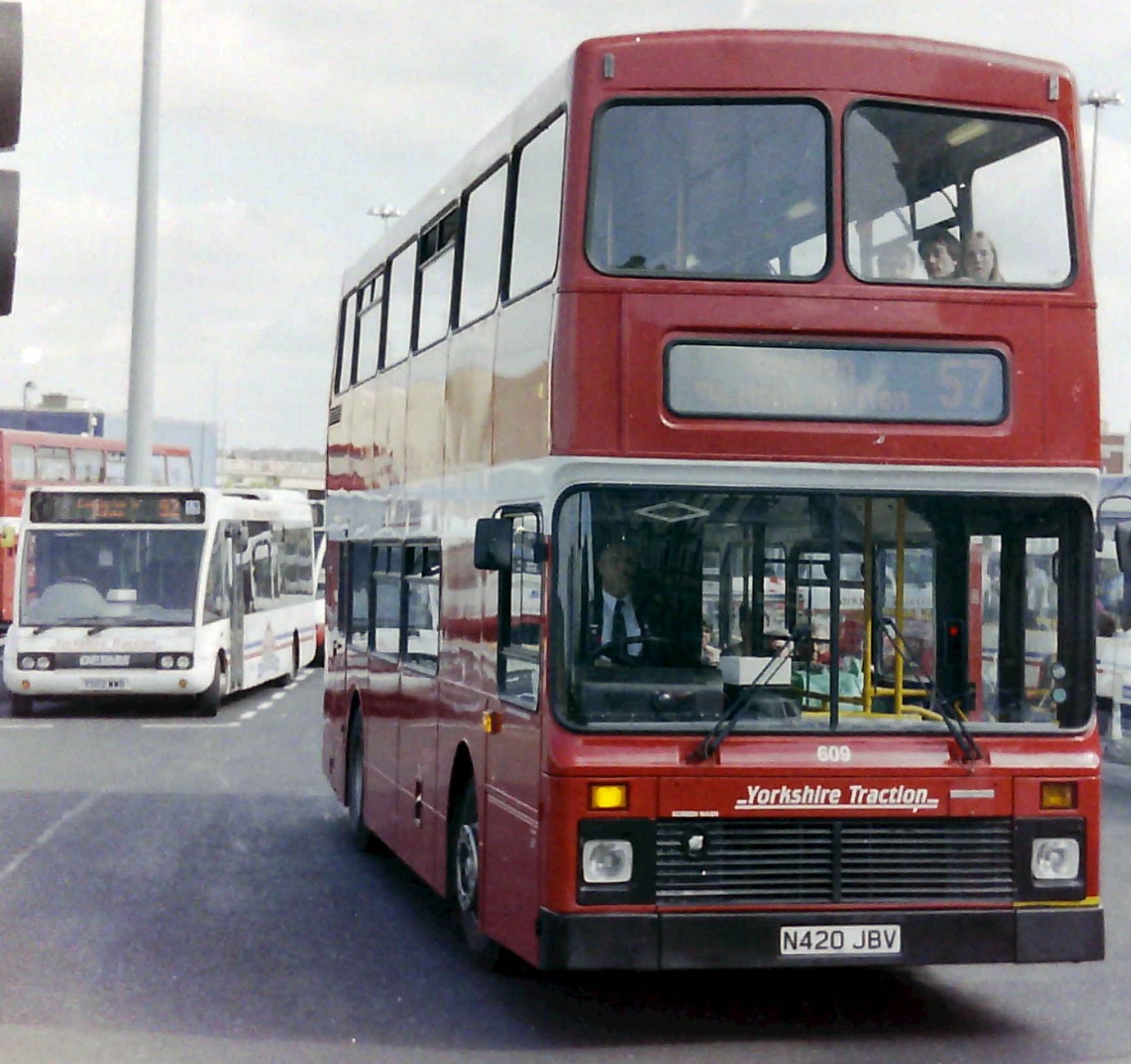The image is a vertical rectangular photograph capturing a bustling bus station scene. Dominating the foreground on the right is a large red double-decker bus with distinctive features. The front of the bus displays the white text "Yorkshire Traction" below the windshield, where the glare makes it difficult to read the destination board, although a red "57" is partially visible. The license plate reads N420JBV. The front upper level, visible through two small windows, shows three seated passengers: a blonde woman, a short-haired brunette man, and an indistinct third individual. The driver, dressed in a white shirt with a black tie and jacket, can be seen through the large lower window, alongside yellow metal handrails near the door. On the left side of the photograph, there's a white single-decker bus and another red double-decker bus in the background. Additionally, the scene includes a glimpse of a tall white building and a standing pole, against a cloudy sky with some sunlight casting shadows on the paved lot below.